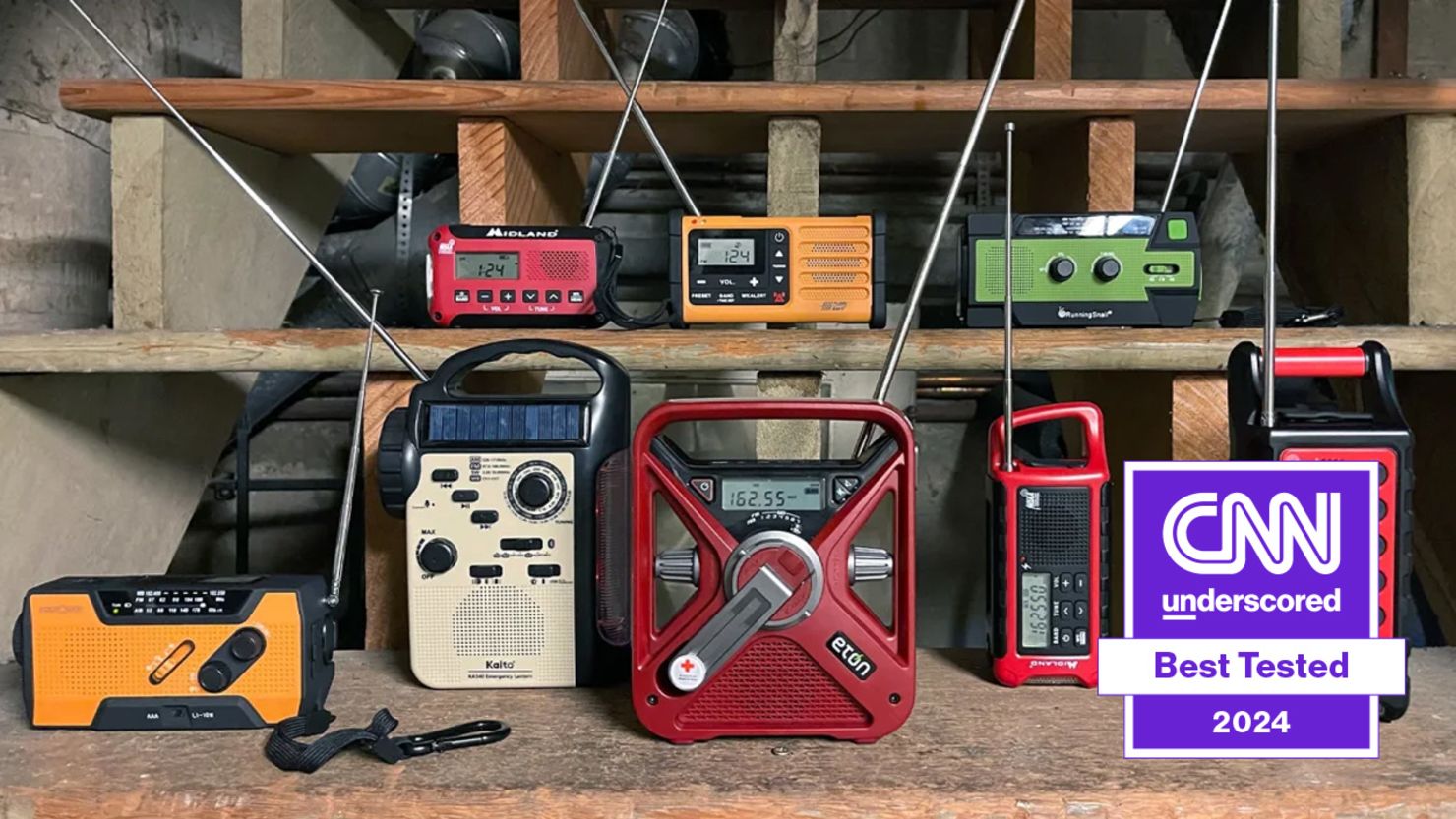The image showcases a collection of vintage, portable transistor radios arranged on dark brown shelves, which appear to be set against cinderblock walls in an old-timey shop. The radios come in a variety of colors, including four red, two orange, one green, and one white, and are notable for their large antennas. Some radios are also mentioned to be on hollow wooden steps, suggesting the image might have been taken in a basement-like setting. Each radio features a dial, underscoring their retro design. In the lower right corner of the image, there's a watermark or graphic banner from CNN Underscored, stating "Best Tested 2024," indicating the photograph may be part of a product review or comparison article.